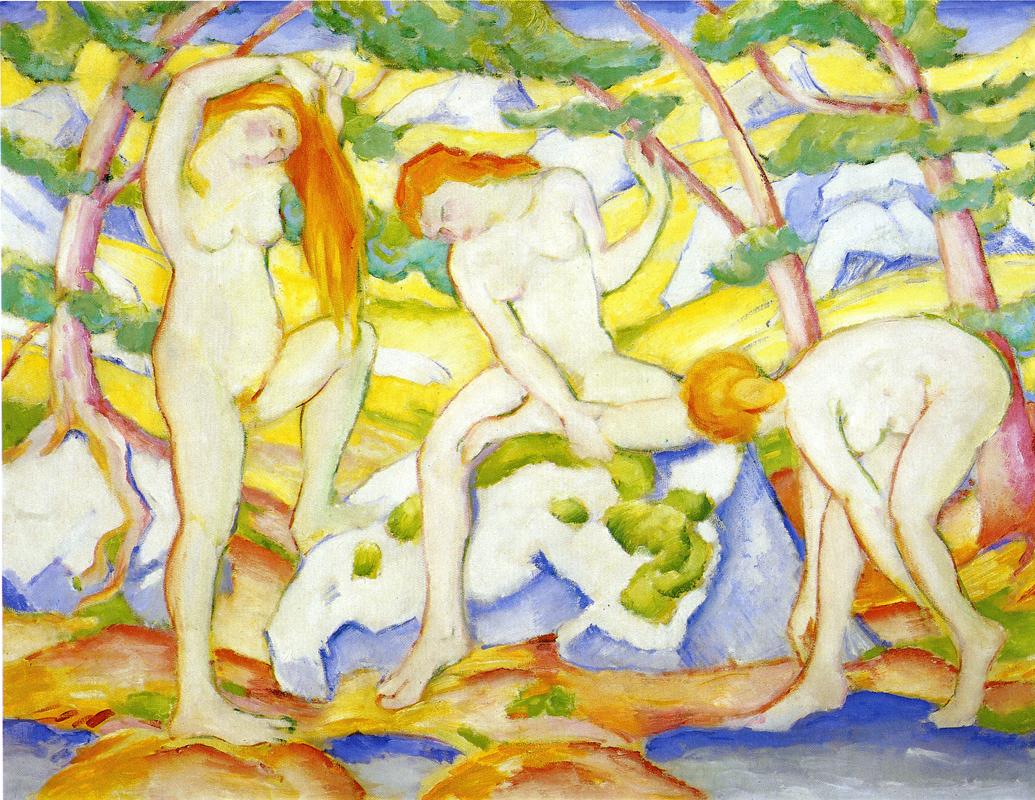This detailed painting, evocative of a style similar to Salvador Dali's dancers, depicts three unclothed women in a serene riverside setting, surrounded by lush trees and vibrant colors. The woman on the left stands gracefully with her right leg perched on a rock, her orange hair cascading as she raises both arms to fix it. The central figure is seated on a rock, her left leg crossed and supported by her right hand, while her left arm reaches upwards, seemingly interacting with a tree branch. The third woman, positioned on the right, is bent over at the river’s edge with both hands near her ankles, perhaps washing herself, her hair tied back. The harmonious blend of indigo blues, greens, yellows, and whites enhance the scene’s tranquility and brightness, capturing a vivid daytime ambiance under a clear blue sky.